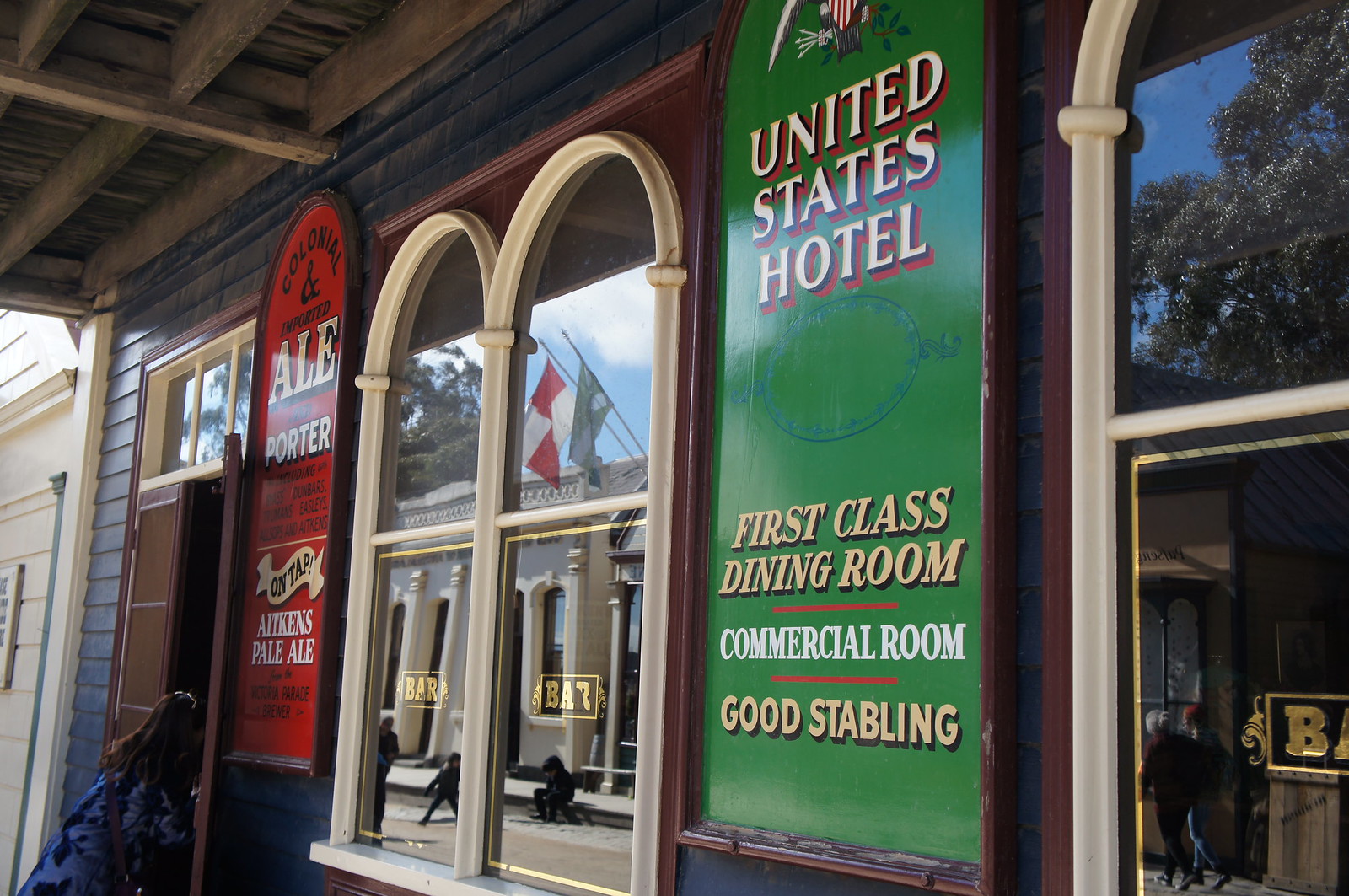The image showcases the exterior of the "United States Hotel," capturing its nostalgic, Old West charm. Prominently displayed on the blue slatted walls are multiple signs, including one green sign that reads "United States Hotel, first-class dining room, commercial room, goods stabling" and another red sign advertising "Colonial and imported ale porter" and "Atkins Pale Ale on tap." The structure features a brown, wooden roof and boasts three large, arched glass windows reflecting the nearby houses. The center window displays the word "Bar" in golden letters. Flanking these windows are smaller ones, with metal bars visible near the rectangular pane to the left of the red sign. A girl in a blue dress is seen entering the door on the left, adding life to the scene. The overall aesthetic and details, such as the reflection of trees and the blue sky, contribute to the vintage saloon-like atmosphere of the hotel.